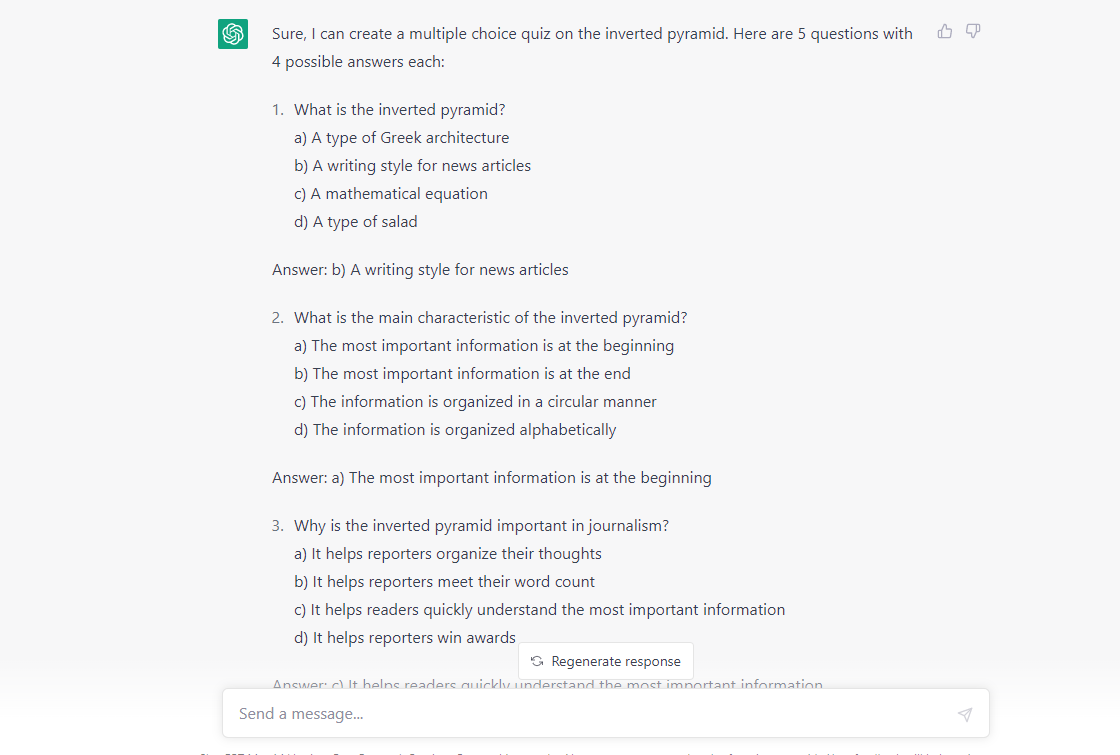The image depicts a conversation interface with ChatGPT, featuring a detailed view of a multiple-choice quiz creation process. In the upper left corner of the interface, there is a distinctive green square, a common visual element in the program's design. The conversation includes numerous questions and corresponding answers.

At the top of the conversation, the user has requested, "Sure, I can create a multiple choice quiz on the inverted pyramid. Here are the five questions with four possible answers each." This introduction suggests that a test pertaining to the "inverted pyramid" is being generated. Adjacent to this question, a thumbs-up and thumbs-down icon are visible, likely allowing for user feedback on the quality of the response.

The visible portion of the quiz displays three clearly numbered questions (1, 2, and 3), each followed by four answer options labeled A, B, C, and D. Although the user indicated there are five questions in total, only three are currently present within the displayed area. The clean layout and structured format of the questions and answers indicate an organized approach to quiz construction.